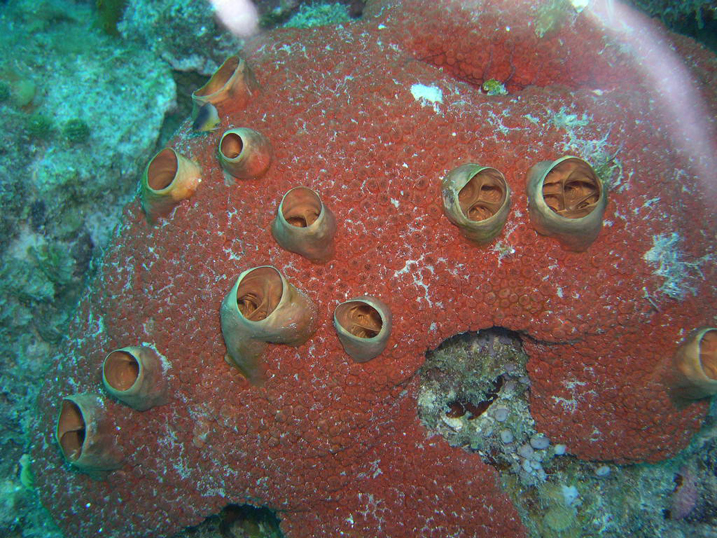In this underwater color photograph, we are peering down at a vibrant, healthy patch of red coral located on a reef. This large, oval-shaped mass spans from the lower left to the upper right of the image and possesses a bumpy, textured surface accentuated with small divots and white patches. The coral itself is predominantly a reddish-pink hue, adding a striking contrast to the surrounding light blue and greenish tones of the rocky sea floor. Scattered across the surface of the coral are numerous oval-shaped, tubular barnacles, appearing sharp and somewhat volcanic. These barnacles, numbering at least ten, are primarily brown with their interiors tinged with orange, and they contribute to the intricate, cave-like details of the coral's structure. Despite being deep underwater, the scene is a close-up view that remains free of any textual elements, highlighting the natural beauty and bustling marine life on this section of the reef.